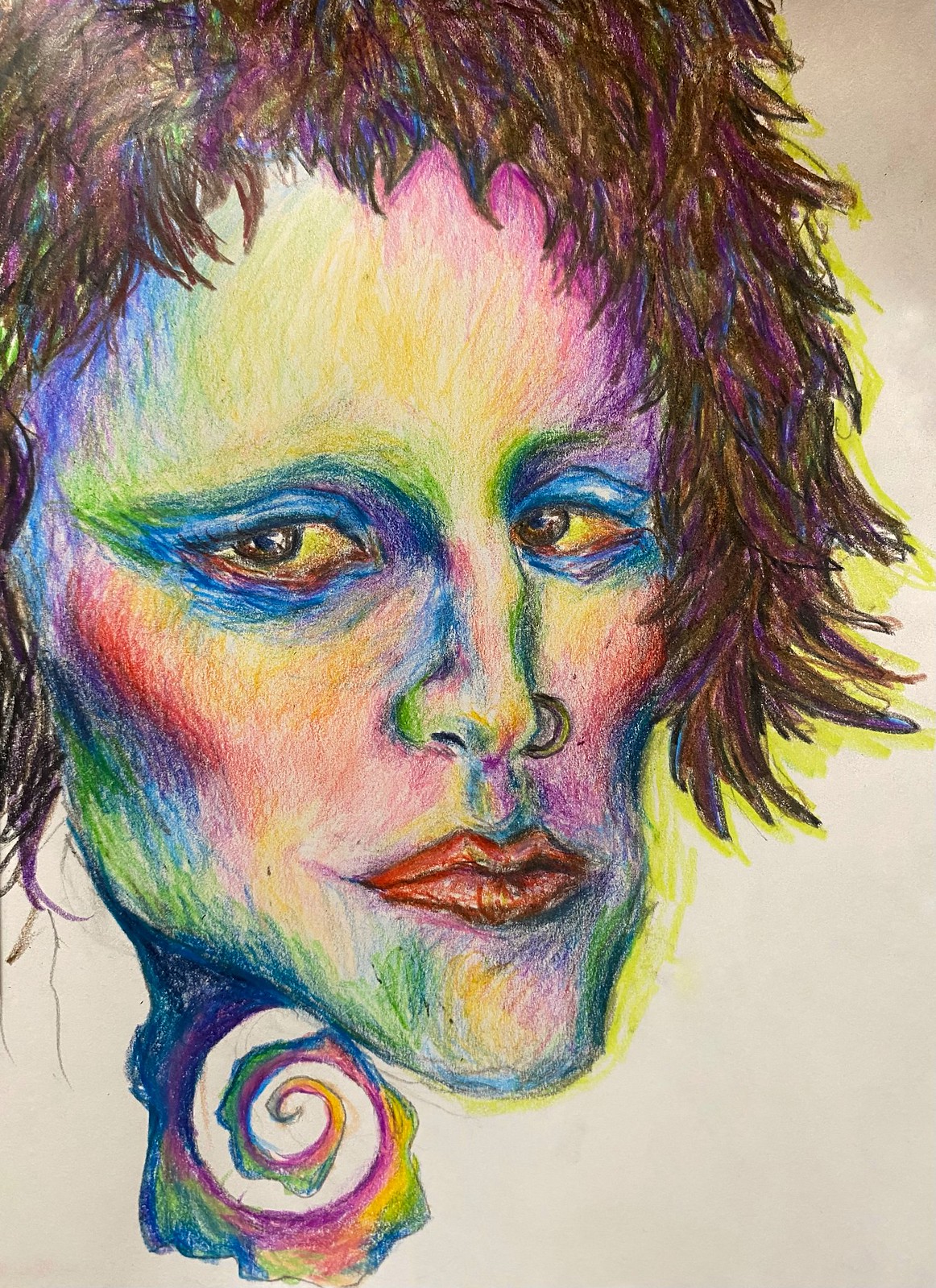This captivating illustration features a vibrant, rainbow-colored face rendered in either colored pencil or acrylics. The subject's face, characterized by high, red-tinged cheekbones and distinct square features, is both striking and expressive. The cheeks appear drawn in, accentuating the sharp contours and high cheekbones. The person has bright red lips and a nose ring, adding fascinating details to their visage. The hair, depicted in jagged strokes of a brownish hue, frames the face dynamically. The eyes, surrounded by blue and green hues, gaze thoughtfully to the left, further enhancing the image's intriguing aspect. Around the face, there are vivid splashes of pink, blue, and green, contributing to the overall rainbow effect. The neck and shoulders of the figure swirl into a white spiral amidst the colorful motif, creating a visually cohesive and mesmerizing piece.